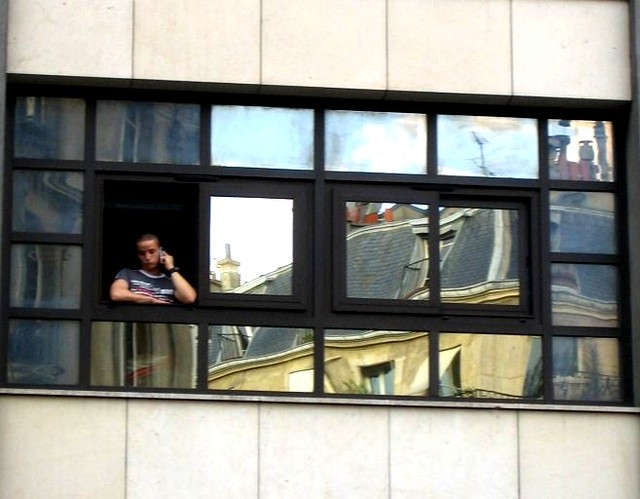In this photograph, we see a striking urban scene centered around a high-up, ornate window, consisting of two sliding central panes bordered by smaller ones, forming an elegant frame. This fancy window belongs to a beige building characterized by large square tiles. Through the leftmost sliding section, which is open, stands a young man with a shaved head, a darker complexion, clad in a gray t-shirt featuring a design on its front. He leans on the outside windowsill with his right arm, while his left arm holds a cell phone to his ear, displaying a serious and focused expression on his face. A watch is visible on his left wrist. The reflective surface of the window captures the image of another building in the distance, suggesting a European architectural style, positioned within a bustling urban environment.